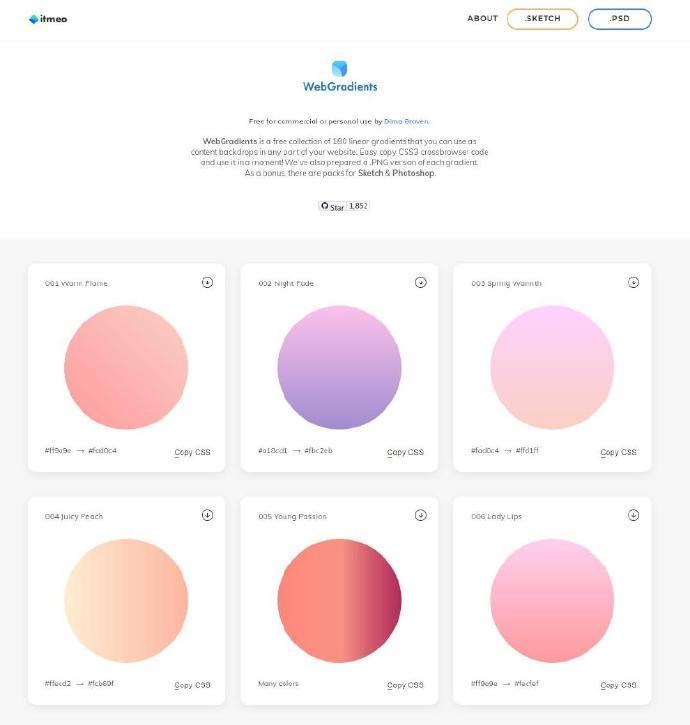The website features a predominantly white background with a light gray bottom section. The top left corner displays the name "ITMEO." To its right are three menu options: "About," "Sketch," and "DSD." Below the menu, the phrase "web gradulence" appears in blue text, accompanied by some exceedingly small black text beneath it.

In the bottom portion of the website, set against the light gray background, are six evenly spaced white squares. Each square contains a large central circle divided into vibrant color segments. The top left segment of the circle is pink, transitioning to purple on the right and a lighter pink further right. The bottom segment is a blend of light beige and pink, while the right half of the circle alternates between red and an orange-pink hue. The rightmost circle segment remains pink.

Each square has a small, slightly illegible name in the top left corner and in the bottom two corners, along with a clock icon in the top right corner.